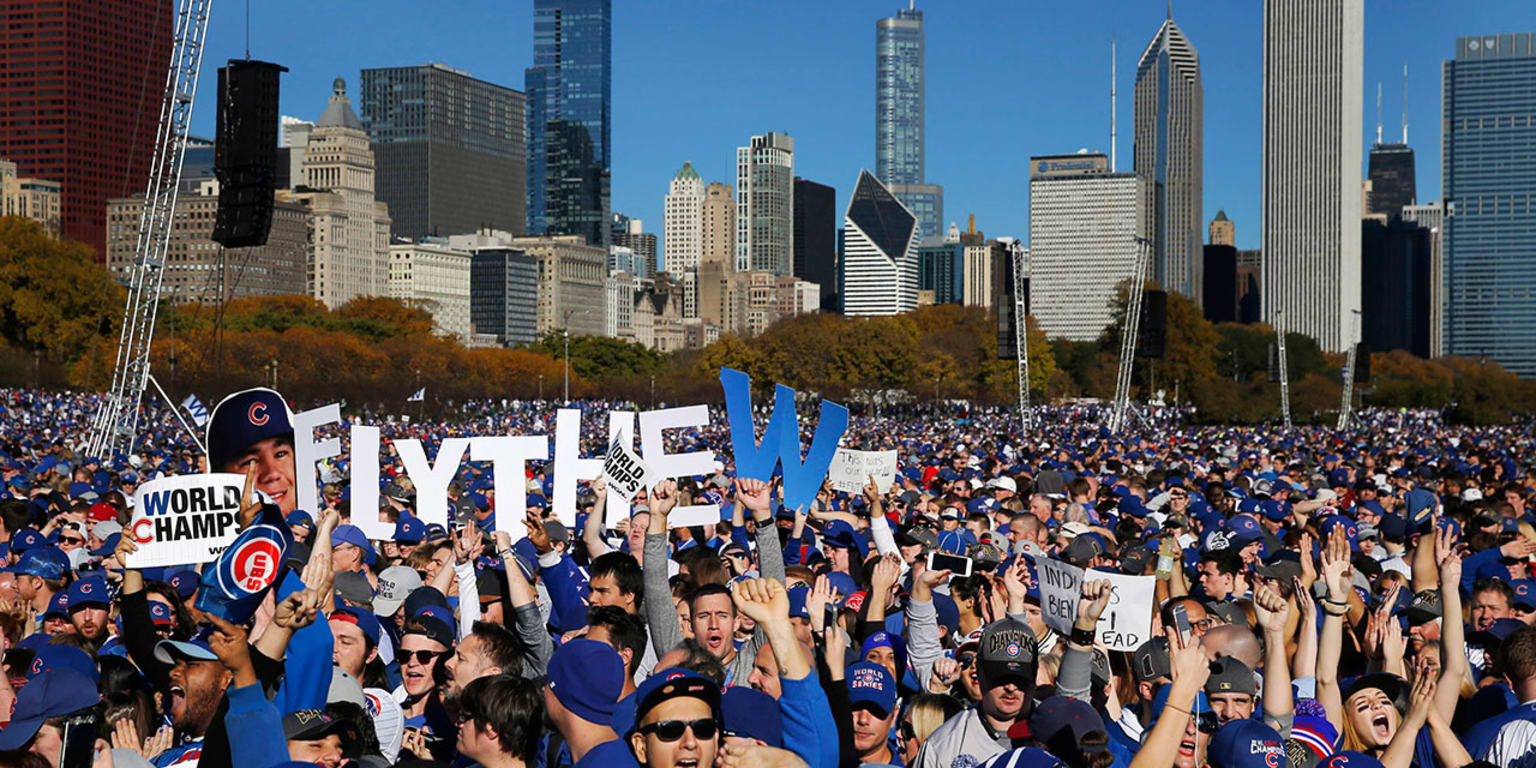The photograph captures an exuberant crowd of Chicago Cubs fans celebrated against a backdrop of a city skyline, likely New York or Chicago, with clear blue skies and numerous skyscrapers. The crowd is adorned in Cubs jerseys, hats featuring the iconic red 'C' logo, and face paint. Their hands are raised in the air as they cheer in unison, creating a lively and joyous atmosphere. Prominently displayed are large letters spelling "Fly the W" in white with a blue 'W', and various signs, including one that reads "World Champs." Additionally, there is a cut-out image of a Cubs player, whose face is held up by the fans, further emphasizing their team spirit and celebratory mood.